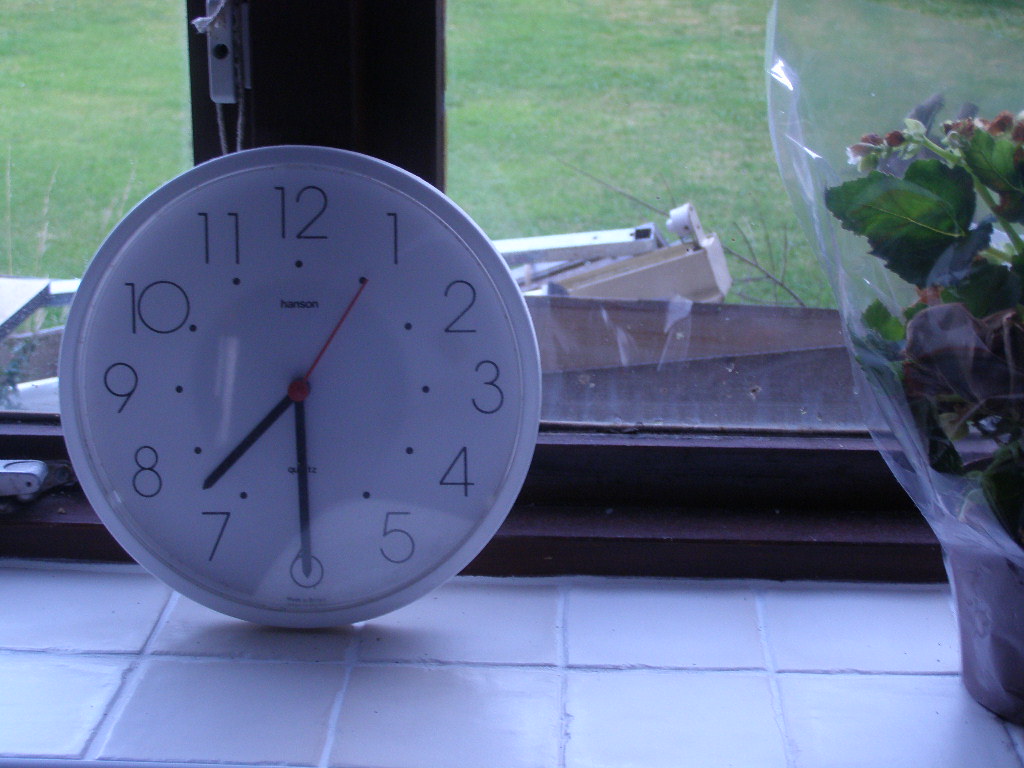This photograph depicts a kitchen countertop featuring a prominent white-rimmed, round, analog wall clock leaning against a window. The clock has a white face, with black numbers from 1 through 12, and small black dots positioned at each numeral. The clock displays the time as 7:30, with black minute and hour hands and a red second hand pointing towards the 1. To the right side of the clock, there is a potted plant with dark soil, green leaves, and red bulbs, enclosed in a sheer plastic wrap. The countertop is made of small, light green square tiles with white mortar. Behind these objects, the window, framed in brown, offers a view of a neatly cut grass lawn with a ladder lying on the ground outside.